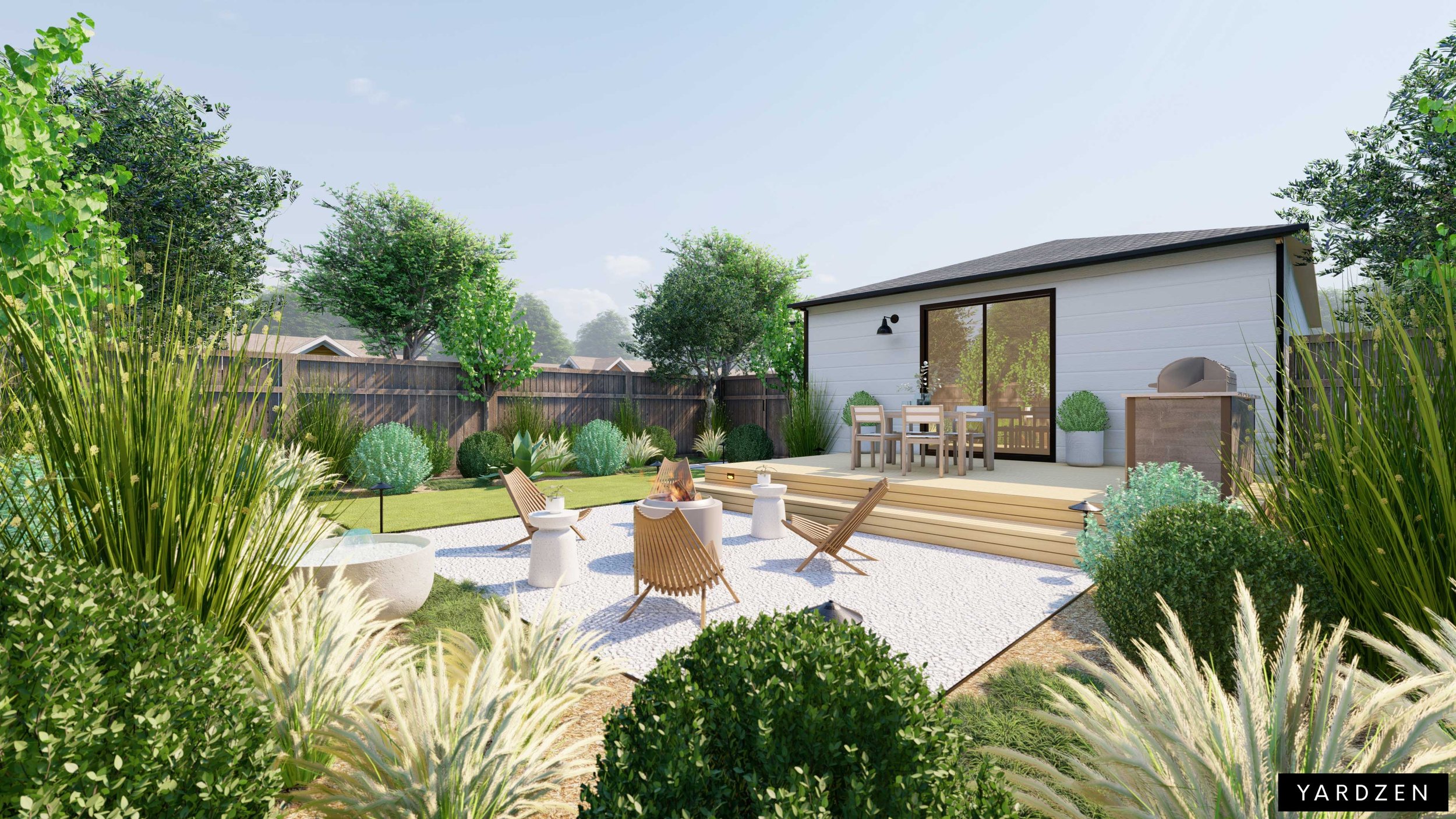This photograph showcases a meticulously manicured backyard with diverse, natural landscaping. A variety of tall green grasses, foxtail grasses, and neatly trimmed, round shrubs create a lush, textured ambiance. At the center of the yard is a square white deck, furnished with assorted brown wooden and wicker-style chairs and featuring a fire pit as the focal point. The yard is enclosed by a wooden privacy fence and dotted with an assortment of trees and native plants of varying shapes and sizes.

The backdrop includes a white house with black accents, equipped with two sliding glass doors each flanked by potted plants, and a black lamp affixed to the exterior wall. A small text in a black box at the lower right corner reads "YARDZEN," hinting at a professional design touch. The overall composition of the scene is both visually appealing and functional, embodying a perfect blend of natural beauty and human-made structure.